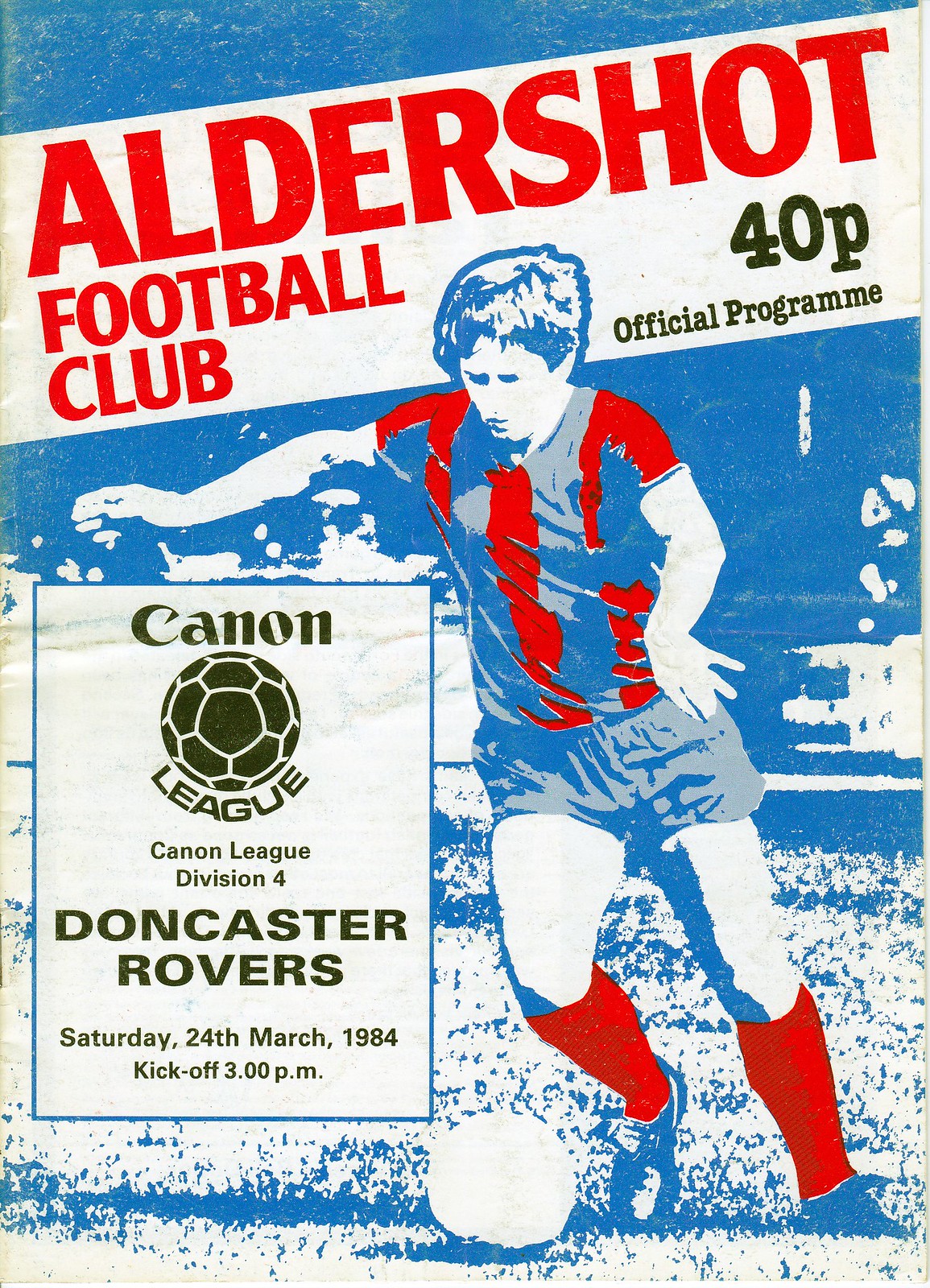This image is the front cover of an official match day program for the Aldershot Football Club. Dominated by hues of blue, red, and white, it features a painting-style sketch of a soccer player in action. The player, wearing a red and blue jersey, red socks, and blue shorts, is depicted running while looking down at a white soccer ball. At the top of the cover, bold red lettering announces "Aldershot Football Club," with "40p Official Program" printed below in black text. The background showcases a blue and white sketch-like depiction of a football field. On the left side of the cover, within a white rectangle, there is black text stating "Canon League Division 4," followed by "Doncaster Rovers." Additional details include the match date, "Saturday, 24th March 1984," and the kickoff time, "3 p.m." This official program vividly combines artistic elements with practical information about the game.